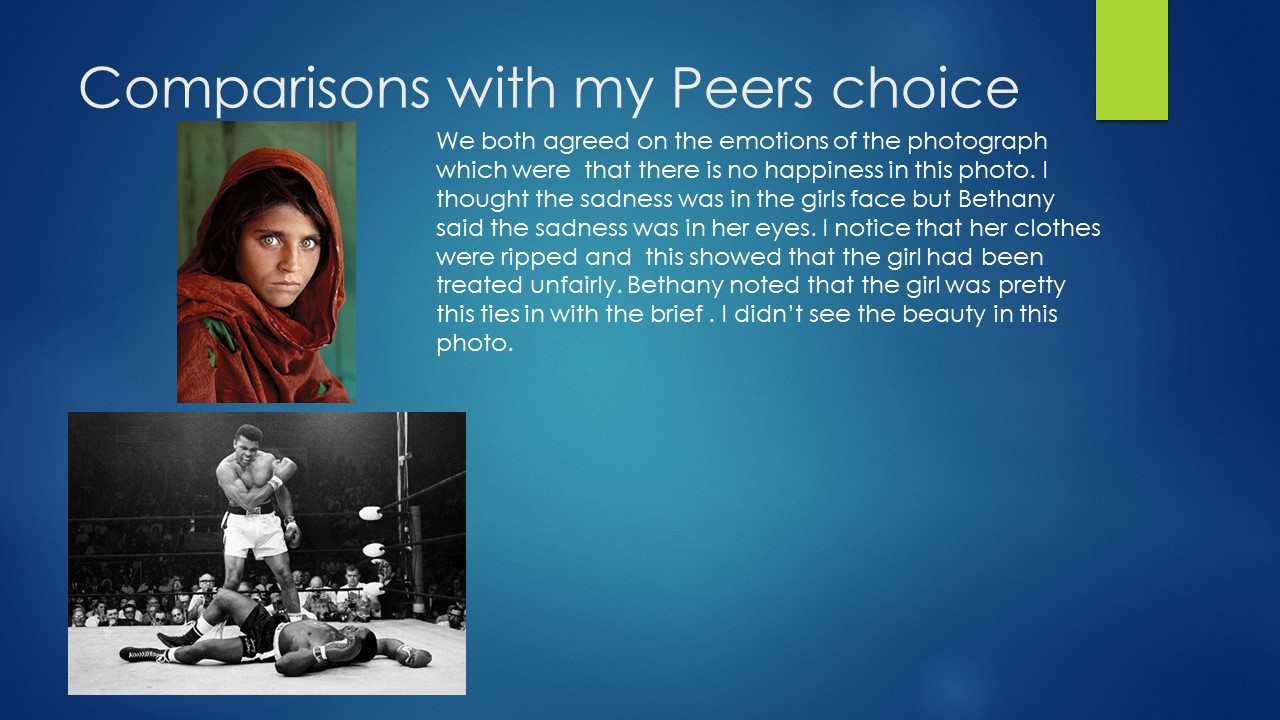This PowerPoint slide, titled "Comparisons with My Peers' Choice," features a detailed comparison between two iconic photographs against a blue, gradient background with dark edges and a lighter center. The left side showcases a famous portrait of a young Afghan girl with striking blue eyes and a red headscarf, expressing sadness. Below it, there's a black and white photograph of Muhammad Ali triumphantly standing over a floored opponent in a boxing ring. A white, sans-serif headline shares the slide’s title, and beneath it, a paragraph in the same white font details an analysis: "We both agreed on the emotions of the photograph, which were that there is no happiness in this photo. I thought the sadness was in the girl's face, but Bethany said the sadness was in her eyes. I noticed that her clothes were ripped, and this showed that the girl had been treated unfairly. Bethany noted that the girl was pretty. This ties in with the brief. I didn't see the beauty in this photo." A lime green rectangle vertically hangs from the top right corner, akin to a digital page marker, adding a pop of contrasting color. This slide blends photographic representationalism with graphic design elements to discuss perceptions of the conveyed emotions within the images.